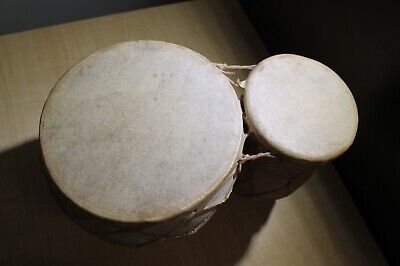The image depicts a pair of bongo drums viewed directly from above. The drums consist of a larger and a smaller cylinder, both covered with a taut, light tan animal hide that shows faint brownish hues due to heavy shadowing. The bongos are connected to each other by some thin strands, making them a unified set. The photograph is in color and shows these drums placed on a smooth, light wooden table, which appears striped with narrow, darker horizontal bars extending to the right due to the shadows cast by the drums. While the sides of the cylinders are obscured by significant shading, the top view highlights the texture and age of the hide, suggesting the drums are quite old, potentially vintage. Overall, the image is fairly dark, with heavy shadows engulfing the sides of the drums and parts of the table.